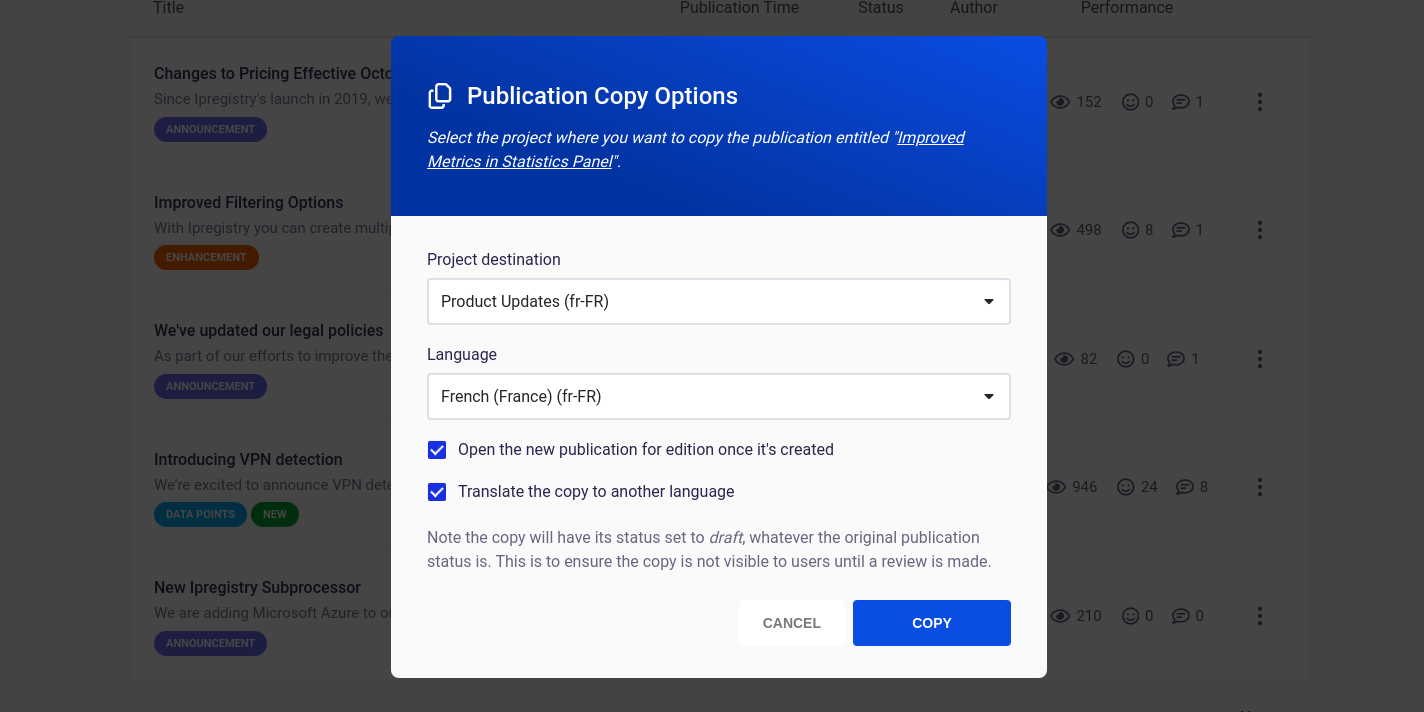The image depicts a user interface screen dedicated to publication copy options. The top section of the screen features a blue background with white text that reads "Publication Copy Options." Below, the background transitions to white, displaying black text labeled "Project Destination" and "Product Updates (FR-FR)." There is a dropdown menu next to "Language" that is set to "French (France) (FR-FR)."

Two blue checkboxes are also visible. The first checkbox is labeled "Open the new publication for editing once it's created," and the second checkbox is labeled "Translate the copy to another language." A note follows, explaining that the translated copy will initially be set to draft status—regardless of the original publication's status. This measure ensures that the copy remains invisible to users until a review is completed. At the bottom of the screen, there is an option to "Cancel Copy." The repeated note emphasizes the importance of the copy being invisible to users until it has been reviewed.